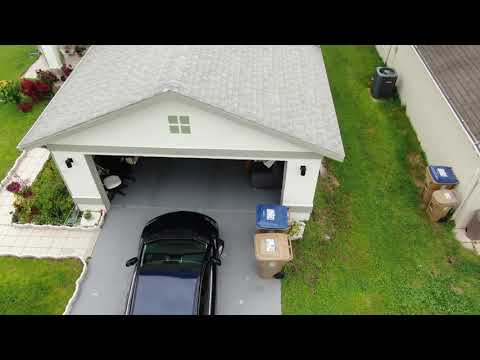The image captures an overhead view of a detached garage with light gray shingle roofing. The garage, whose wide door is open, reveals a car parked on the edge of the driveway. Above the door, there is a gray line running horizontally, topped by a window with four panes. On the right side of the car, two trash cans are positioned—one blue and one light brown. The left side of the driveway features a walkway that angles back towards the top-left of the image. Surrounding the garage structure on both sides is green grass. To the right, the side of another white building with a brown roof is visible, adjacent to additional trash cans—one brown and one brown with a blue lid—and an air conditioner in the upper right corner. The photo appears to be taken from a slightly upward tilt angle, providing a comprehensive view of the scene.